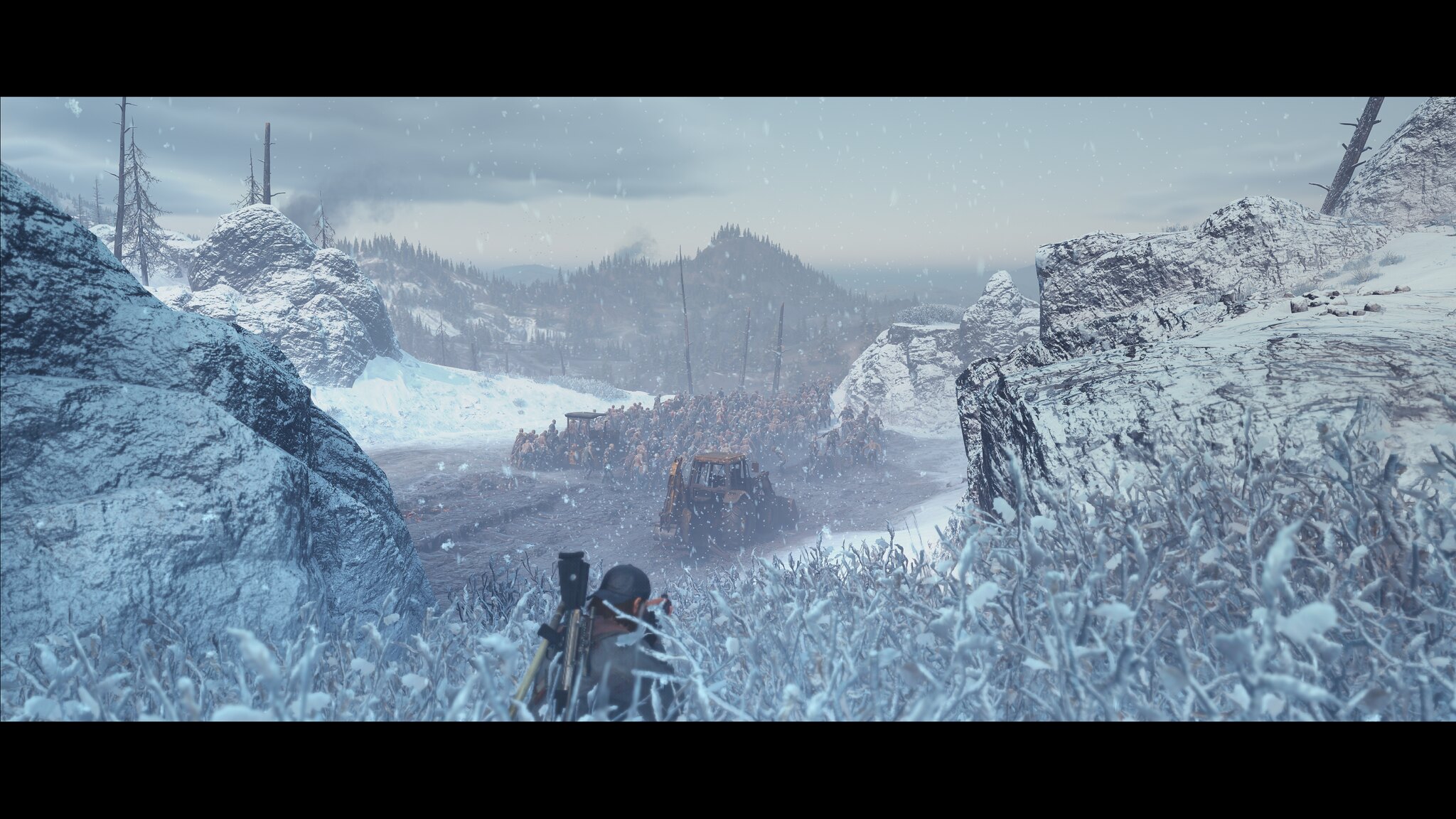A mesmerizing screenshot from an unidentified video game captures an immersive third-person perspective of a snowy outdoor setting. Delicate snowflakes are gently falling, adding to an already thick blanket of snow covering the rugged terrain, suggesting the scene is set in a high-altitude or mountainous region. In the distance, a small flat area can be seen, featuring what appears to be cultivated crops alongside a lone tractor, indicating an isolated farming endeavor amid the harsh environment. The protagonist is portrayed in a crouched position within the dense, knee-high grass, closely observing the tranquil, yet intriguing landscape.